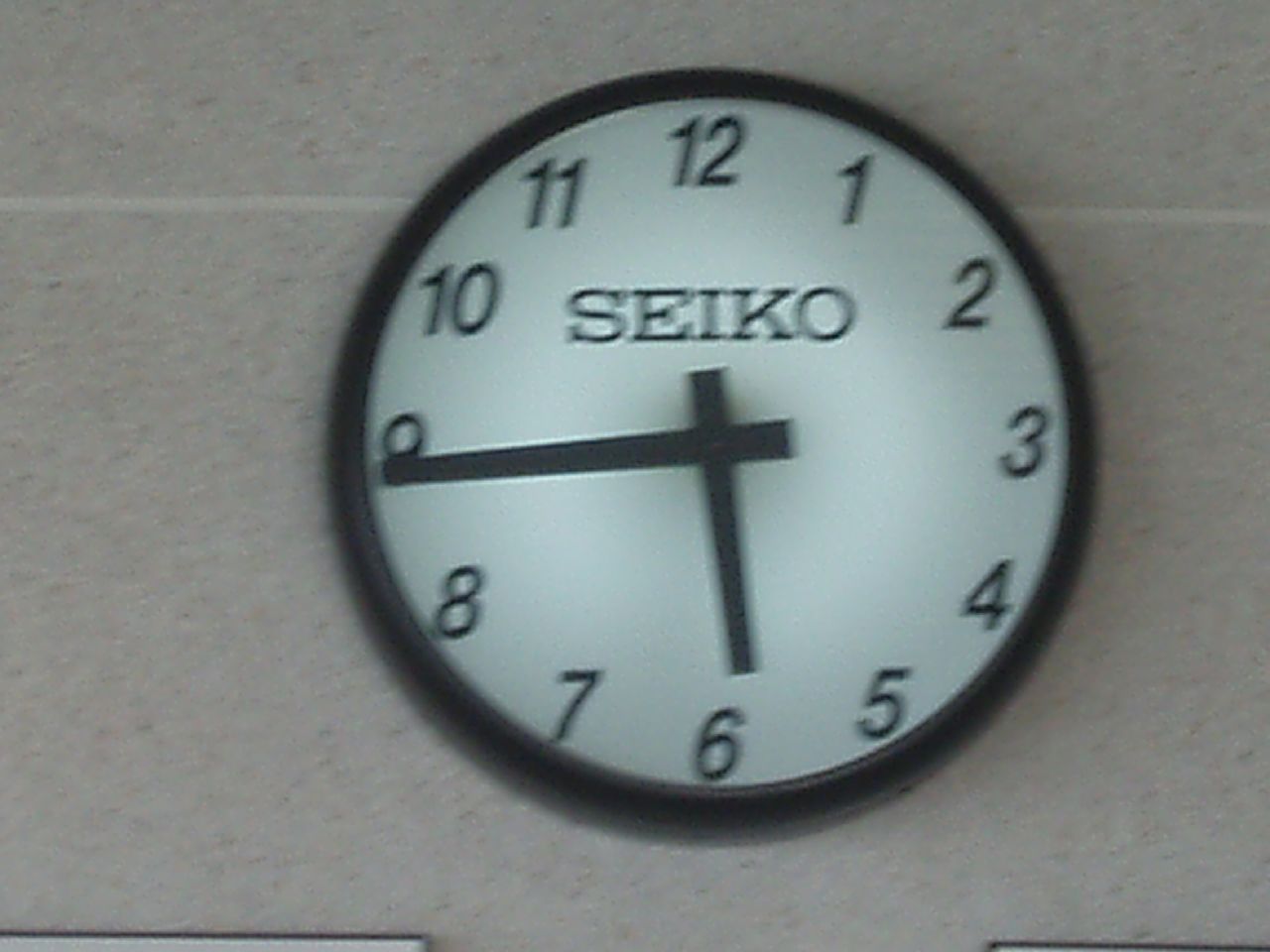The image depicts a classic wall clock with a minimalist design. Centered on the clock's clean, white face are bold black numbers ranging from 1 to 12, ensuring easy readability. Prominently positioned near the center, the brand name "SEIKO" is displayed in uppercase letters. The clock features two substantial, rectangular-shaped hands for the minute and hour indicators. Encasing the clock is a simple, sleek black frame that contrasts sharply with the background. The setting of the clock is a textured stone wall, giving it a rustic backdrop. Towards the top of the clock, remnants of grout or adhesive can be seen, suggesting it may have been recently mounted or repositioned. At the very bottom edge of the image, two tiny, indistinct objects are visible, adding a slight element of curiosity to the scene.